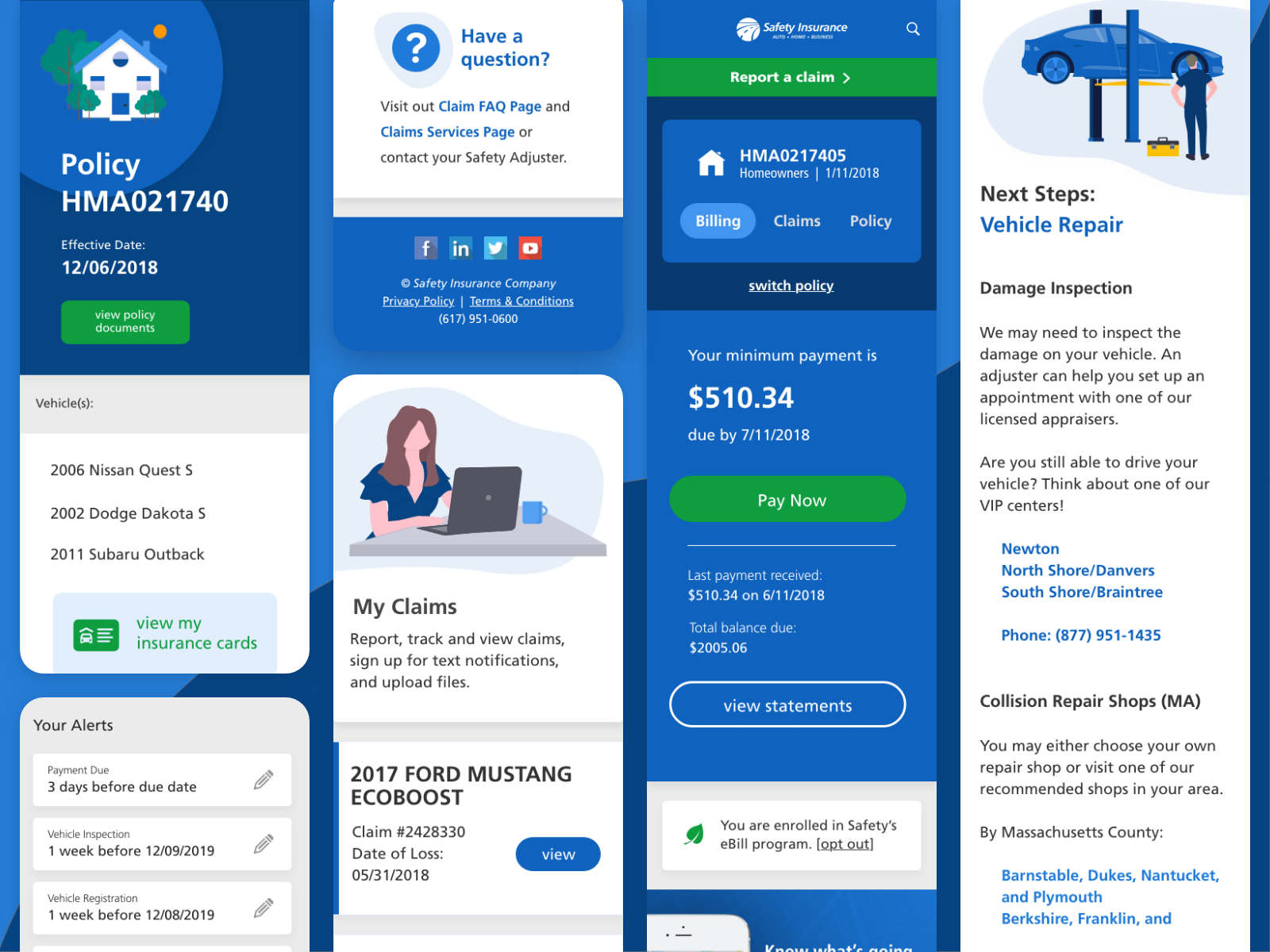The on-screen image appears to be a detailed interface of a vehicle auto insurance policy. The screen predominantly features blue and white colors. 

**Upper Left Section:**
- A cartoon-style illustration of a house with a green tree and an orange sun. 
- Below this, the word "Policy" is displayed in white.
- Additional text follows: "HMA 021740."
- Below this, in smaller font, it says "Effective Date: 12/06/2018."
- A green button below reads "view policy documents" in lowercase white font.

**Policy Details:**
- A white box with a gray header labeled "Vehicles(s):"
- Lists three vehicles:
  - 2006 Nissan Quest
  - 2002 Dodge Dakota
  - 2011 Subaru Outback
- A light blue box with green text that says "view my insurance cars," with a small gray box to the left.

**Alerts Section:**
- Gray box labeled "Your Alerts."
- Displays three white rows with various alerts:
  - Payment due three days before due date with a pencil icon.
  - Vehicle inspection one week before 12/09/2019 with a pencil icon.
  - Vehicle registration one week before 12/08/2019 with a pencil icon.
- A blue circle with a white question mark and the text "Have a question?" to the right.
- Below this, it states "Visit our Claim FAQ page and Claim Services page or contact your Safety Adjuster," with "Claim FAQ page," "Claim Services page," and "Safety Adjuster" capitalized and in blue text.

**Social & Company Information:**
- Icons for Facebook, Instagram, Twitter, and YouTube.
- Contact and policy information:
  - "Safety Insurance Company Privacy Policy Terms and Conditions" followed by the phone number "617-951-0600."

**Claim Details Section:**
- A white box featuring a cartoon woman with long hair on a laptop.
- Text reads "My Claims Report: Track and view claims, sign up for text notifications, and upload files."
- Another box specifies:
  - "2017 Ford Mustang EcoBoost"
  - "Claim Number: 2428330"
  - "Date of Loss: 05/31/2018"
  - A blue "view" button.

**Footer Section:**
- A blue row that states "Safety Insurance" at the top.
- A green bar with "Report a Claim" in white with a right arrow icon.
- Another house illustration labeled "HMA 0217405."
- "Homeowners 1/11/2018" followed by "Billing Claims Policy."
- A "Switch Policy" link in white.
- Payment information:
  - "Your minimum payment is $510.34 due by 7/11/2018."
  - A green "pay now" button.
  - "Last payment received $510.34 on 6/11/2018."
  - "Total balance due $2,005.06."

**E-Bill Program:**
- A white box stating "You are enrolled in Safety's e-bill program" with the option to "opt out."

**Next Steps:**
- On the right, an icon of a car on a jack with a mechanic.
- "Next Steps" in black text with "Vehicle Repair" in blue:
  - "Damage inspection" in black.
  - Instructions for vehicle damage inspection and contact details for setting up an appointment with an adjuster.
  - Inquiry if the vehicle is still drivable, with information about VIP centers in Newton, North Shore/Danvers, South Shore/Braintree.
  - Contact information: "877-951-1434 / 1435."
  - "Collision repair shops in MA (Massachusetts)" with counties listed (Barnstable, Dukes, Nantucket, Plymouth, Berkshire, Franklin, etc.).